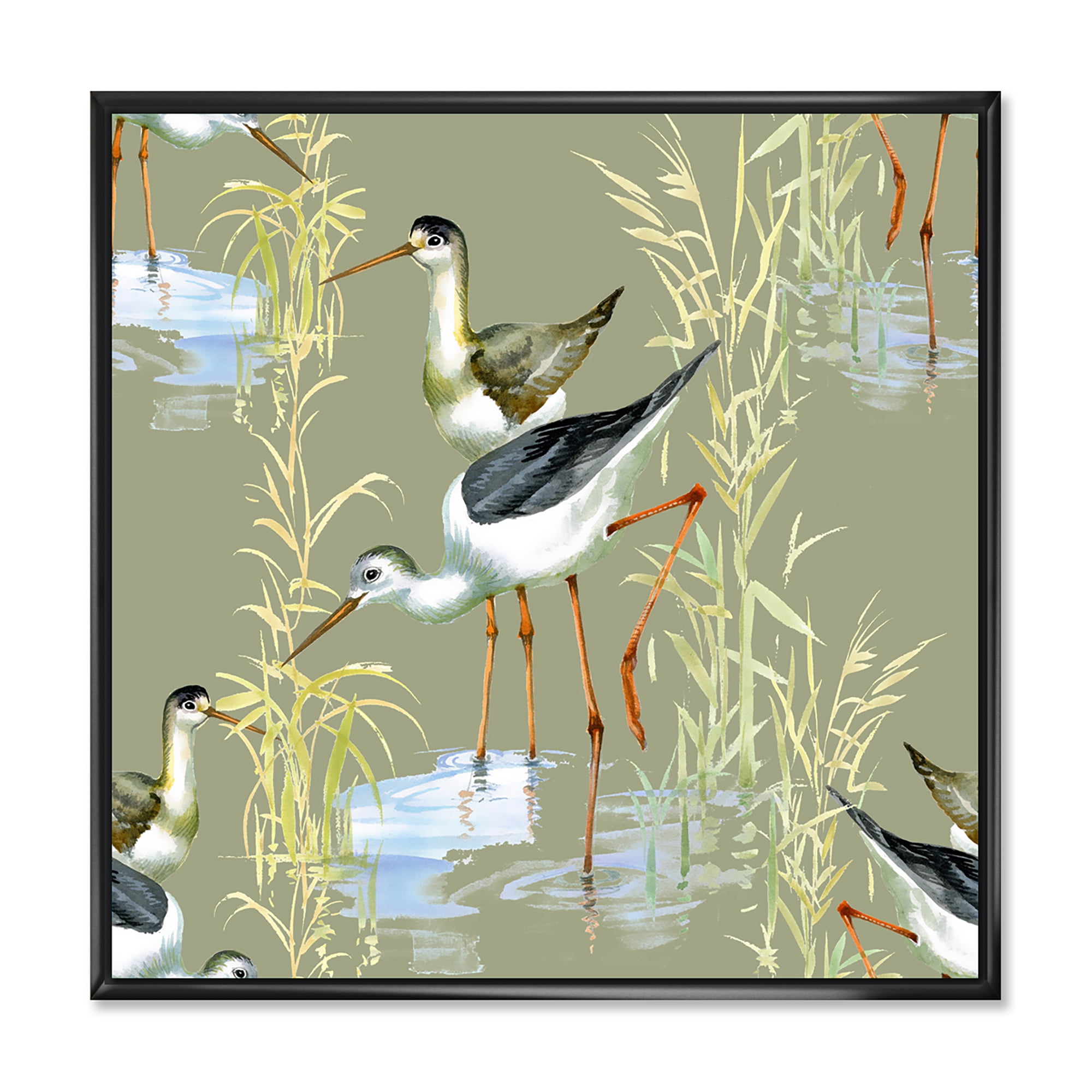The image is a detailed painting of a wildlife scene, framed with a thin black outline, likely square in shape. The painting depicts an aquatic environment, featuring a group of tall, long-legged birds standing in swampy water. The water appears dark with a tannish-green hue, while blue rippled puddles form around the birds' legs. The foreground is filled with yellowish-green grass sprouting from the water, creating a dynamic natural setting.

In the center of the painting, two birds are fully visible, showcasing elongated orange legs and pointy orange beaks. Their bodies are primarily white, with some having black or dark brown wings. Additional birds are partially visible around the edges, displaying body parts such as necks, backs, legs, and tail feathers. Some birds also exhibit different colorations, including light brown heads and blackish markings on their top feathers. Other colors present in the painting include tan, beige, sage green, light blue, and hints of wood orange and white.

The overall composition suggests a lively but serene outdoor setting, meticulously crafted to capture the essence of wetlands teeming with bird life.